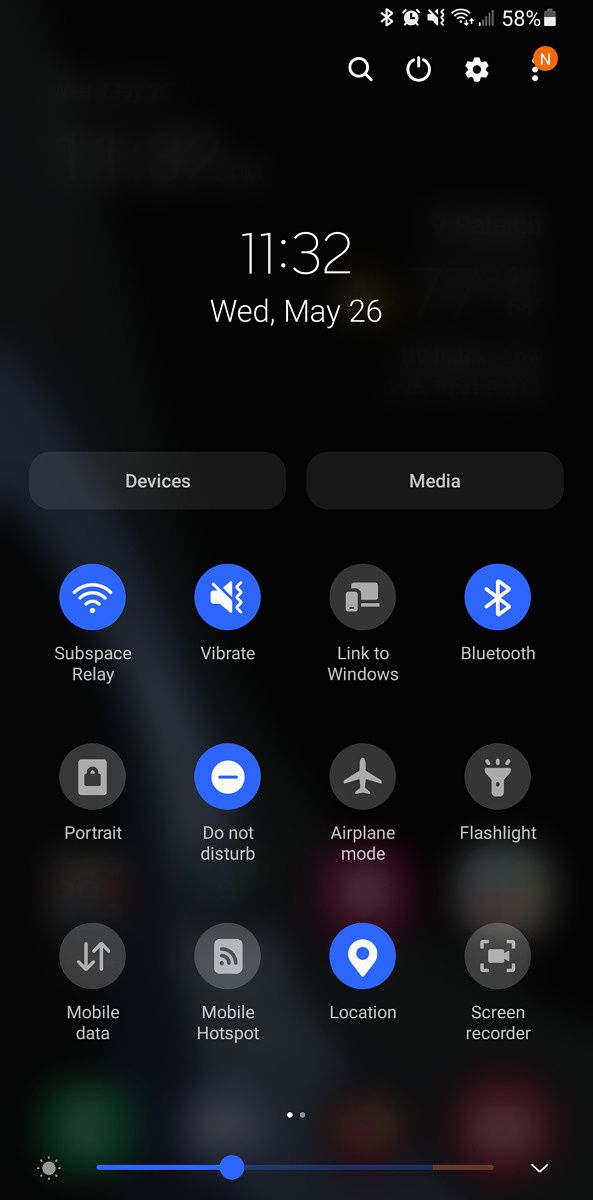In this image, set against a solid black background, the top portion displays a status bar with a battery indicator at 58%, a magnifying glass icon, a clock, and a settings icon. Additionally, there are three dots with a red dot containing the letter 'N.' Below this, the screen shows the time as 11:32 AM on Wednesday, May 26. Two prominent buttons labeled "Devices" and "Media" are featured, alongside various icons representing functions like Subspace, Subspace Relay, Vibrate, Link to Windows, Bluetooth, Portrait, Do Not Disturb, Airplane Mode, Flashlight, Mobile Data, Mobile Hotspot, Location, and Screen Recorder. Towards the bottom of the image, there's a small gray dot, followed by a gradient line transitioning from blue to red. A manipulable blue dot on the gradient line allows user interaction. Additionally, there are two small white dots, followed by a down arrow, completing the detailed interface.